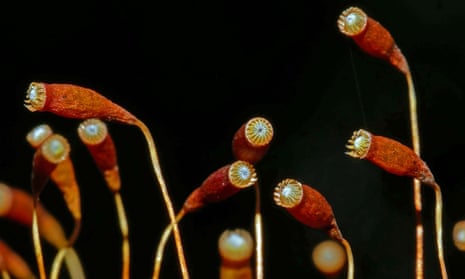This image is a small, rectangular photograph, roughly three inches wide by two inches high, featuring a curious and unusual type of flower or weed. The background is a deep brownish-black, providing a stark contrast to the main subjects. Rising up from the bottom of the image, there are about ten long, narrow stems, each approximately an eighth of an inch wide. These stems, a brownish color, splay out in various directions, with some appearing head-on while others are viewed from the side.

Topping each stem is a rounded, tubular structure, around a quarter of an inch wide and extending up to half an inch in length. These tubular shapes are a striking reddish-orange hue with a reddish band near the tip. Beyond this band, the tubular ends feature small yellow spikes or teeth with silvery-gray centers and a black dot at the core, giving them an almost plug-like appearance.

Some of the tubular flowers at the bottom of the image appear blurred, emitting a glow similar to headlights. The effect adds to the abstract quality, making them seem to shine. The entire image bears an eerie resemblance to a mix of flowers and microphone cords, contributing to the overall enigma of what type of plant this might be.